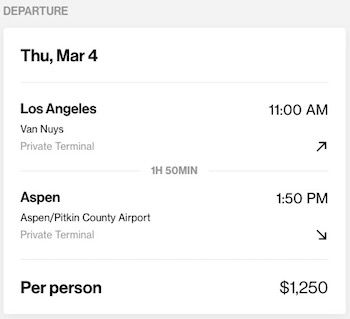This image displays a cropped screenshot of a departure section from an airline booking. The background is grey at the top left corner with the word "DEPARTURE" prominently displayed in capital letters in a dark grey font. Below this, a large white box contains detailed flight information.

At the top left of the white box, the departure date is indicated as "Thursday, March 4th" with a small grey line underneath separating it from the airport details. The airport of origin is listed as "Los Angeles, Van Nuys," with a note below it that says "private terminal" in light grey font. On the right side, the departure time is specified as "11:00 AM" accompanied by an arrow pointing upwards to the right.

Further down, another thin grey line separates this segment from additional details, including flight duration and arrival information. In the center of this line, it is stated that the flight duration is one hour and 50 minutes. Below this, on the left side, the destination is noted as "Aspen, Aspen-Pitkin County Airport, private terminal." On the right side, the arrival time is listed as "1:50 PM" with an arrow pointing down to the left.

Below these details, the pricing information is included. It states "per person" in large black font on the left, and the cost "$1250" on the right. This departure section is cropped from the main body of the flight information.